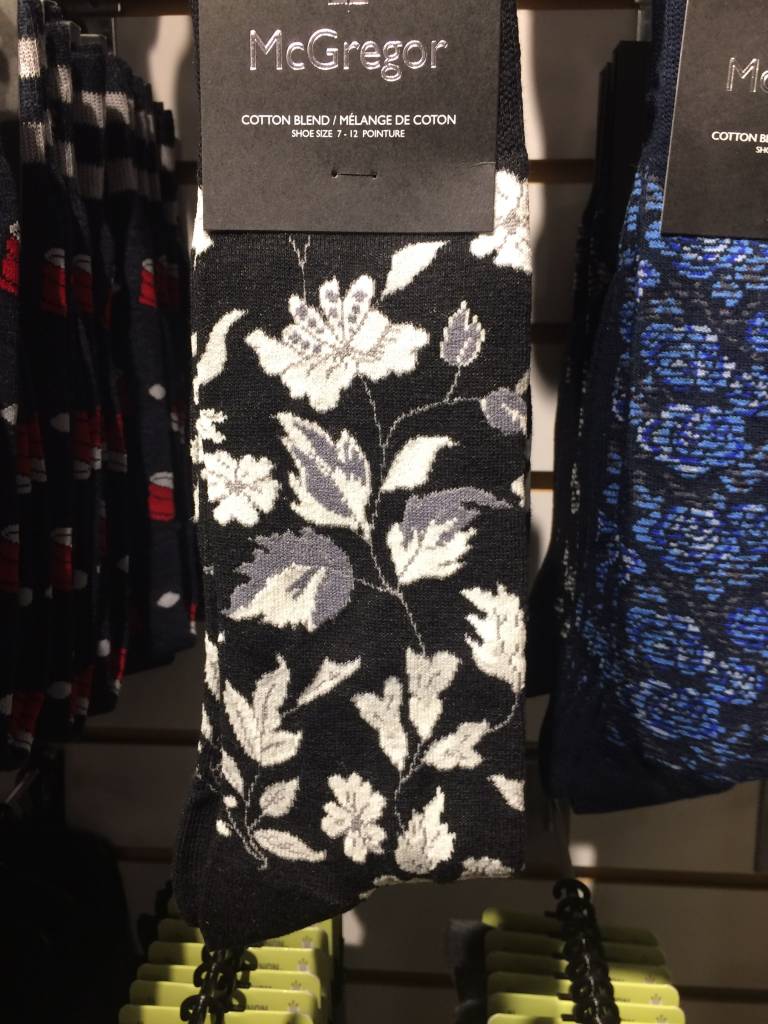This is a full-color, vertically rectangular photograph taken indoors at a clothing store, focusing on a retail display of socks. At the bottom of the image, two rows of socks hang on hooks, each with yellowish price tags. Above these, three pairs of socks are prominently displayed in a row. The left pair is predominantly black with red and white accents. The center pair features a black body adorned with a floral pattern in white and gray; its black label reads "McGregor Cotton Blend," indicating it fits shoe sizes 7 through 12. The right pair of socks also has a black body, decorated with blue flowers. The photograph highlights the variety in design and color while emphasizing the brand's details on the label.